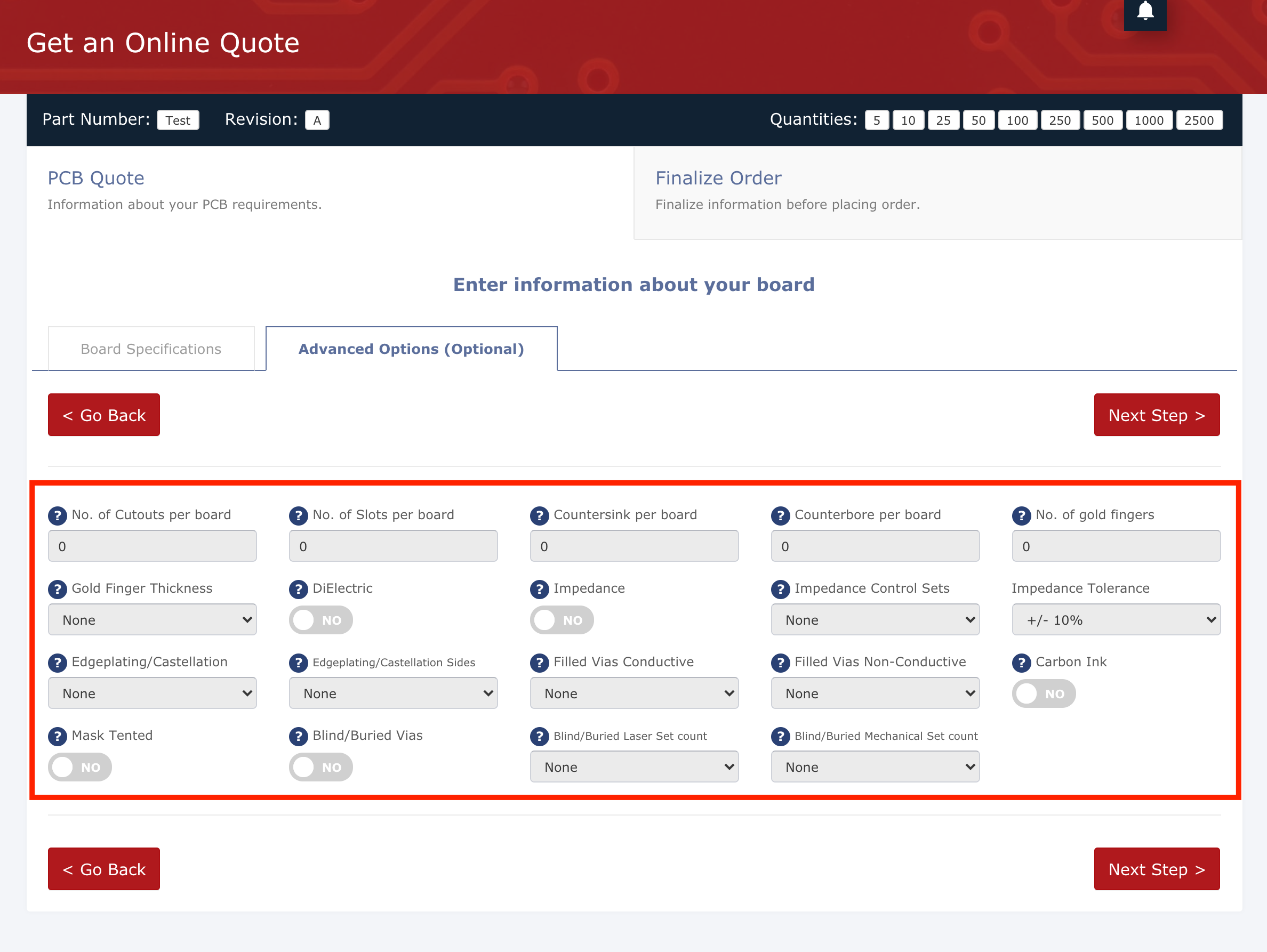The image depicts an online platform dedicated to obtaining quotes for PCB (Printed Circuit Board) manufacturing, although the specific website name is unclear due to the absence of a visible web address bar or company branding.

At the top of the page, a prominent red header reads: "Get an Online Quote - Part Number, Test Revision A." Below this, there is a dropdown menu to select quantities, ranging from 5 to 2,500 units.

Moving to the center of the page, an area titled "PCB Quote" details the steps for specifying PCB requirements and finalizing the order. There are two primary sections for entering information: one for board specifications and another for advanced options, currently highlighted in blue.

The lower-middle portion of the interface outlines several customizable options for the PCB, all set to default values of zero or 'no.' Options include:
- Number of cutouts per board: 0
- Number of slots per board: 0
- Countersinking per board: 0
- Counter boring per board: 0
- Number of gold fingers: 0
- Gold fingers thickness
- Dielectric
- Impedance
- Impedance control sets
- Impedance tolerance: ±10%
- Edge plating and castellation (including sides)
- Filled vias – both conductive and non-conductive
- Carbon ink: No
- Mask tinting: No
- Blind and buried vias: No
- Blind buried laser set count: None
- Blind buried mechanical set count: None

At the bottom, there are red buttons for navigation: "Next Step" to proceed with the order and "Go Back" options for revisiting previous steps. The overall setup suggests a user interface designed for configuring large-scale PCB manufacturing orders, likely intended for industrial or heavy manufacturing applications.